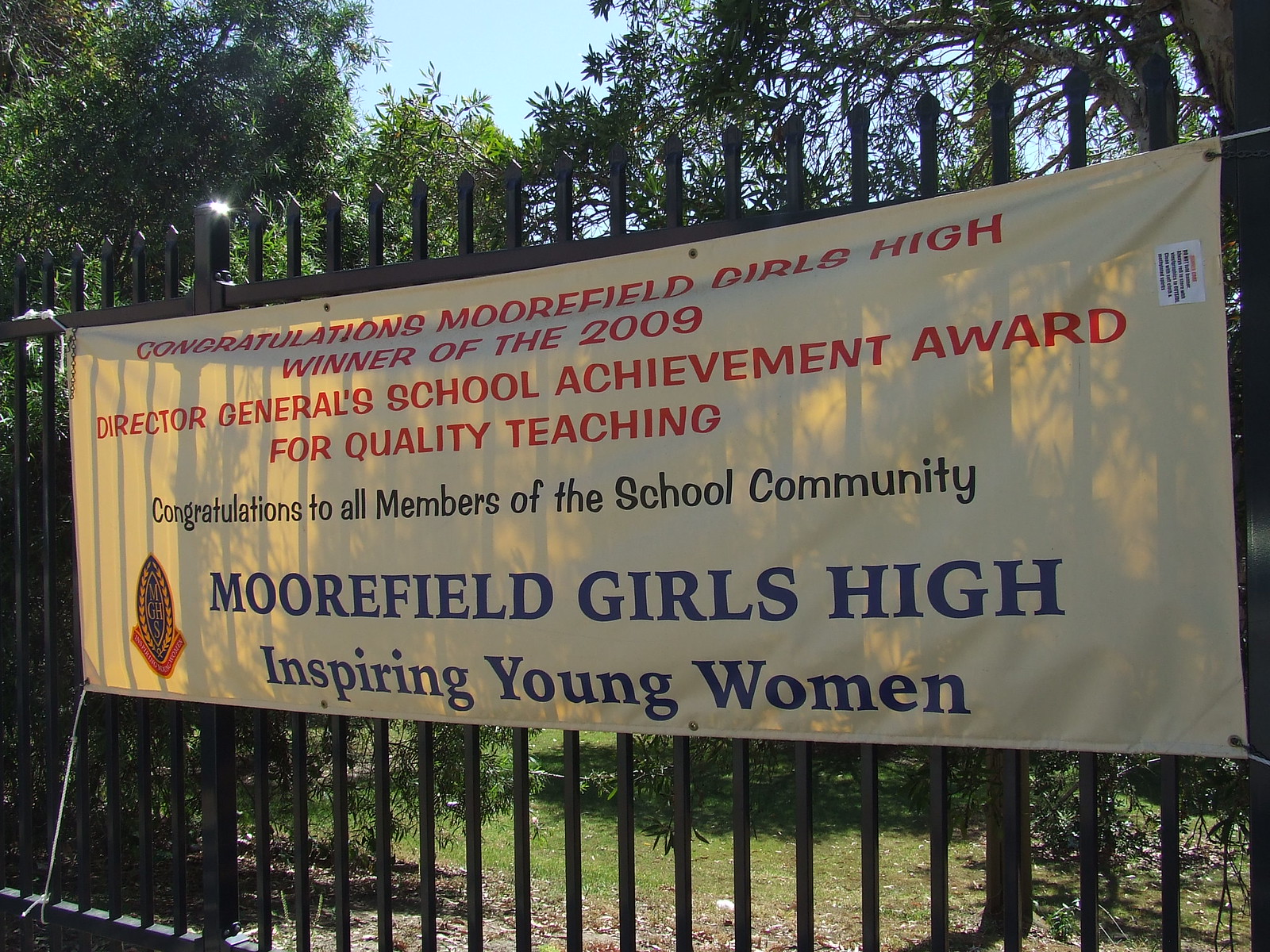The image is a color, daylight, outdoor photograph capturing a bright sunny day with a clear blue sky. Tall, leafy trees serve as a lush backdrop. A large black metal fence, topped with tall, pointed posts, stands prominently in the scene. Attached to the fence with white ties and ropes is a white vinyl sign, slightly transparent to light.

Emblazoned across the top of the sign in bold red capital letters, it reads: "CONGRATULATIONS MOORFIELD GIRLS HIGH WINNER OF THE 2009 DIRECTOR-GENERAL'S SCHOOL ACHIEVEMENT AWARD FOR QUALITY TEACHING." Beneath this, in black font, the sign continues: "Congratulations to all members of the school community." The message concludes in blue text: "Moorfield Girls High Inspiring Young Women," where "Moorfield Girls High" is all capitalized, while "Inspiring Young Women" capitalizes only the initial letters of each word.

Prominently featured on the left side of the sign is an oval-shaped symbol in blue and orange with touches of yellow, resembling a logo. The entire scene is framed by a small patch of grass, enhancing the outdoor setting.